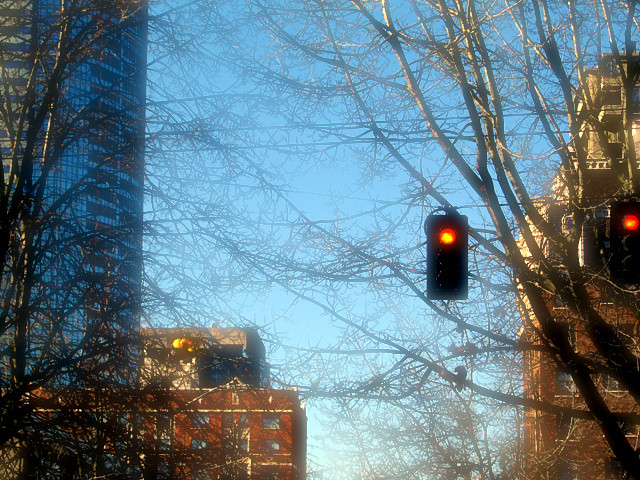In this photograph of an urban scene, two overhead traffic lights are prominently featured, both showing red and suspended from wires that stretch across the frame from left to right. The lights are positioned on the right side of the image. The background reveals a variety of buildings, creating a layered cityscape. Dominating the left side is a towering glass skyscraper with numerous windows, indicative of a high-rise office building. In front of it stands a shorter, red brick building, and behind, partially obscured, is a tan building. 

On the right, more red brick buildings, possibly apartments, can be seen extending from the bottom to the top of the frame. Leafless trees with spindly branches crisscross the scene, their outlines stark against a sky that transitions from light blue at the bottom to a deeper shade as it ascends. The sky occupies a significant portion of the middle and top of the image, adding an element of openness to the urban landscape. The perspective of the photograph tilts slightly upward, emphasizing the verticality of the buildings and the trees, while also giving a glimpse of power lines that support the hanging traffic lights.